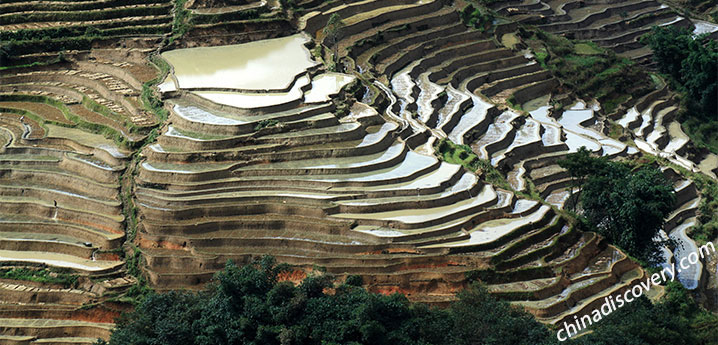This detailed image captures a stunning landscape of terraced rice paddies carved into a mountain, forming a natural staircase design. Each stepped terrace is filled with dark, reflective water that highlights the intricate structure of these rice fields. The organic shape of the terraces follows the natural contours of the land, creating a harmonious blend with the surrounding environment. Around the bottom of the terraced hillside, lush green trees and bushes add a vibrant touch of nature to the scene. The photograph, likely taken from a high vantage point such as a drone or helicopter, offers a broad, sweeping view of this rural farming area, typical of certain regions in China. The bottom right corner of the image bears the text "Chinadiscovery.com" in white font, indicating the location. Notably, the landscape is devoid of any people, emphasizing the tranquil and pristine beauty of the terraced fields.